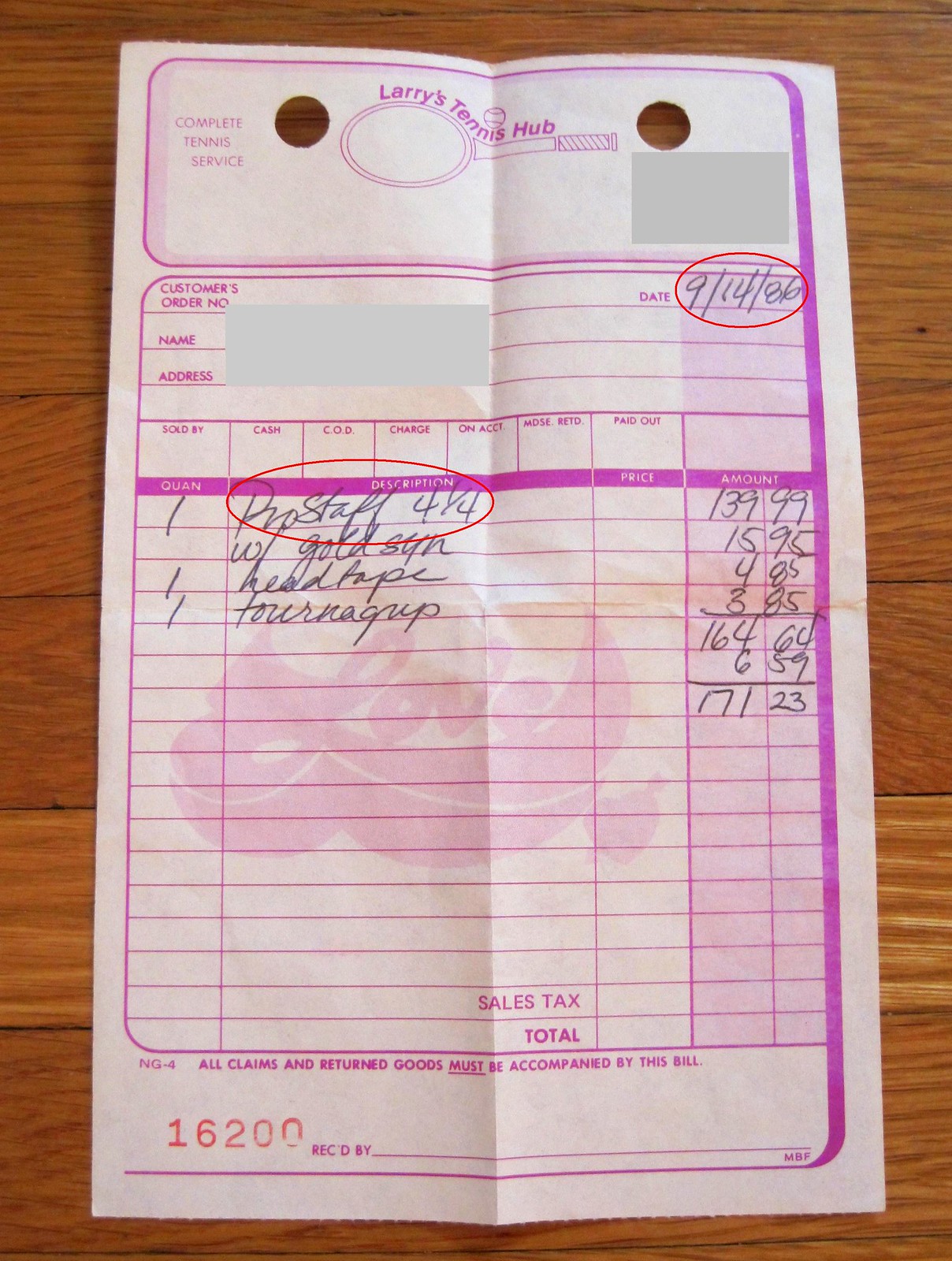This is an image of a receipt from Larry's Tennis Hub. The receipt is white with a purple border, featuring a tennis racket and a tennis ball used creatively to dot the "i" in "tennis." It has two holes on either side where it was attached to a notepad. The customer's order details, including the number, name, and address, are obscured by a white strip of paper. The date on the receipt is September 14, 1986.

The itemized list includes:
- Quantity: Pro Staff 4 1/4 at $139.99
- Gold SYN at $15.95
- One Head Tape at $4.85
- One Turn Grip at $3.85

The subtotal comes to $164.64, and with tax amounting to $6.59, the total is $171.23. The text is printed in black ink, and both "Pro Staff 4 1/4" and the date are circled in red. Additionally, there is a whimsical touch with the word "LOVE" written in bubble letters and a heart pierced by an arrow, all in purple.